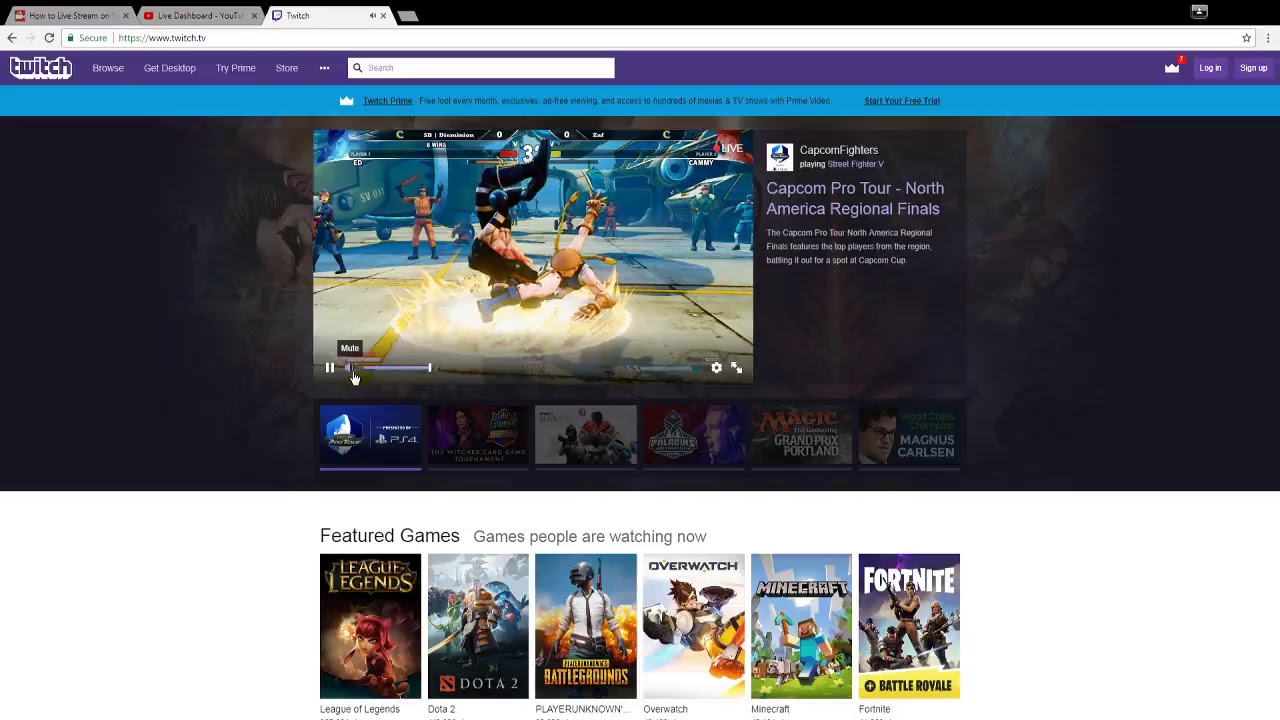This is a detailed screenshot of a web browser with three open tabs, with the active tab being the third one that displays the Twitch website (twitch.tv). The URL bar confirms the website address. Across the top of the screen, there's a prominent purple navigation bar. On the top left corner of this bar, the Twitch logo is visible, rendered in white and purple with a white drop shadow.

In this navigation bar, there are three primary navigation buttons along with four menu items. A white search bar is also present. On the far right side of this bar, you'll find a crown icon followed by two purple buttons reading "Log In" and "Sign Up" with white text.

Central on the screen below the navigation bar is a video stream showcasing a side-scrolling fighting game. To the right of this video, there's text indicating that the event is the "Capcom Pro Tour North American Regional Finals".

Below the video section, there is a section titled "Featured Games," which displays six images of different games.